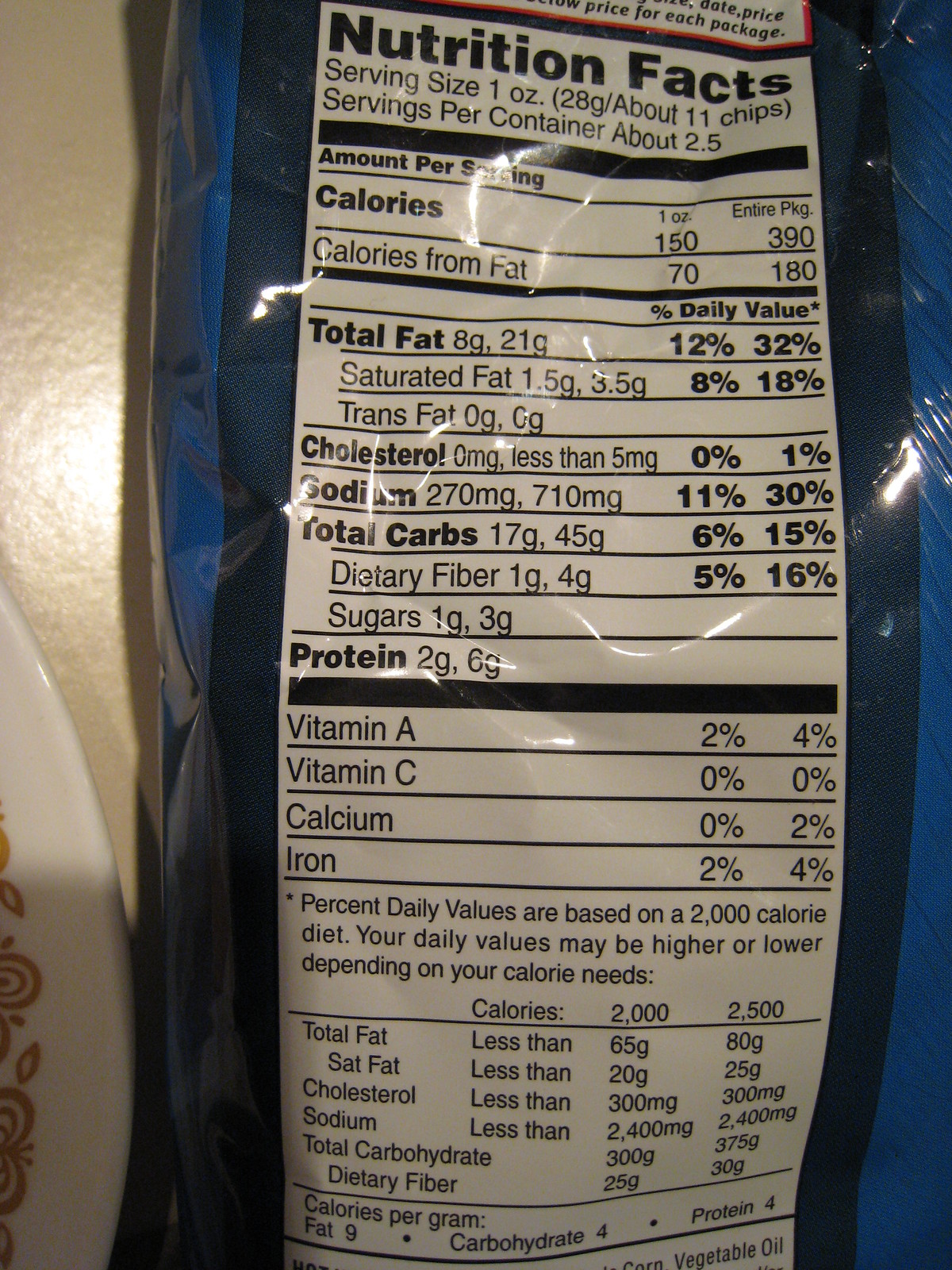An informative look at the nutrition facts displayed on the backside of a blue potato chip bag reveals essential dietary details for consumers. Each serving size is defined as approximately 11 chips or 28 grams. The bag contains about 2.5 servings. A single serving provides 150 calories, culminating in 390 calories for the entire package, aligning perfectly with the indicated servings per container.

In addition to calorie content, the bag details the fat content, cholesterol, sodium, carbohydrates, dietary fiber, and protein levels per serving. Specifically, it lists the following nutritional values: 
- Vitamin A: 2%
- Vitamin C: 0%
- Calcium: 0%
- Iron: 2%

The bag's design features a dark blue background framing the gray 'Nutrition Facts' logo and associated information. The scene is set on a light-colored surface, and a decorated plate is partially visible, peeking out from the left side of the image, adding an elegant touch to the overall composition.